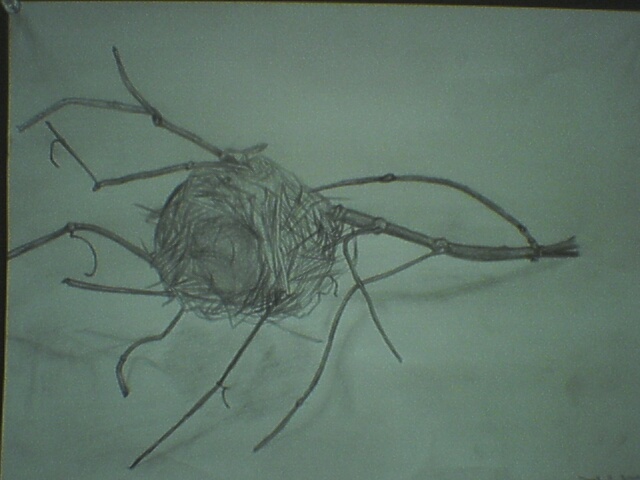This detailed pencil sketch, set against a horizontal white sheet of paper, artistically captures a small tree branch with several twigs extending from it. The branch is positioned with its thickest, broken-off end at the right center of the image, while the thinner twigs radiate towards the center and left-hand side. Attached to the branch is a somewhat spherical object, likely representing either a beehive or a bird's nest. This feature is rendered with numerous long, curved, and twisted lines, forming a large, lightly shaded mass that contrasts with the finer details of the twigs. The artist's meticulous pencil work brings a sense of texture and depth to the composition, highlighting the intricate interplay between nature's forms and textures.